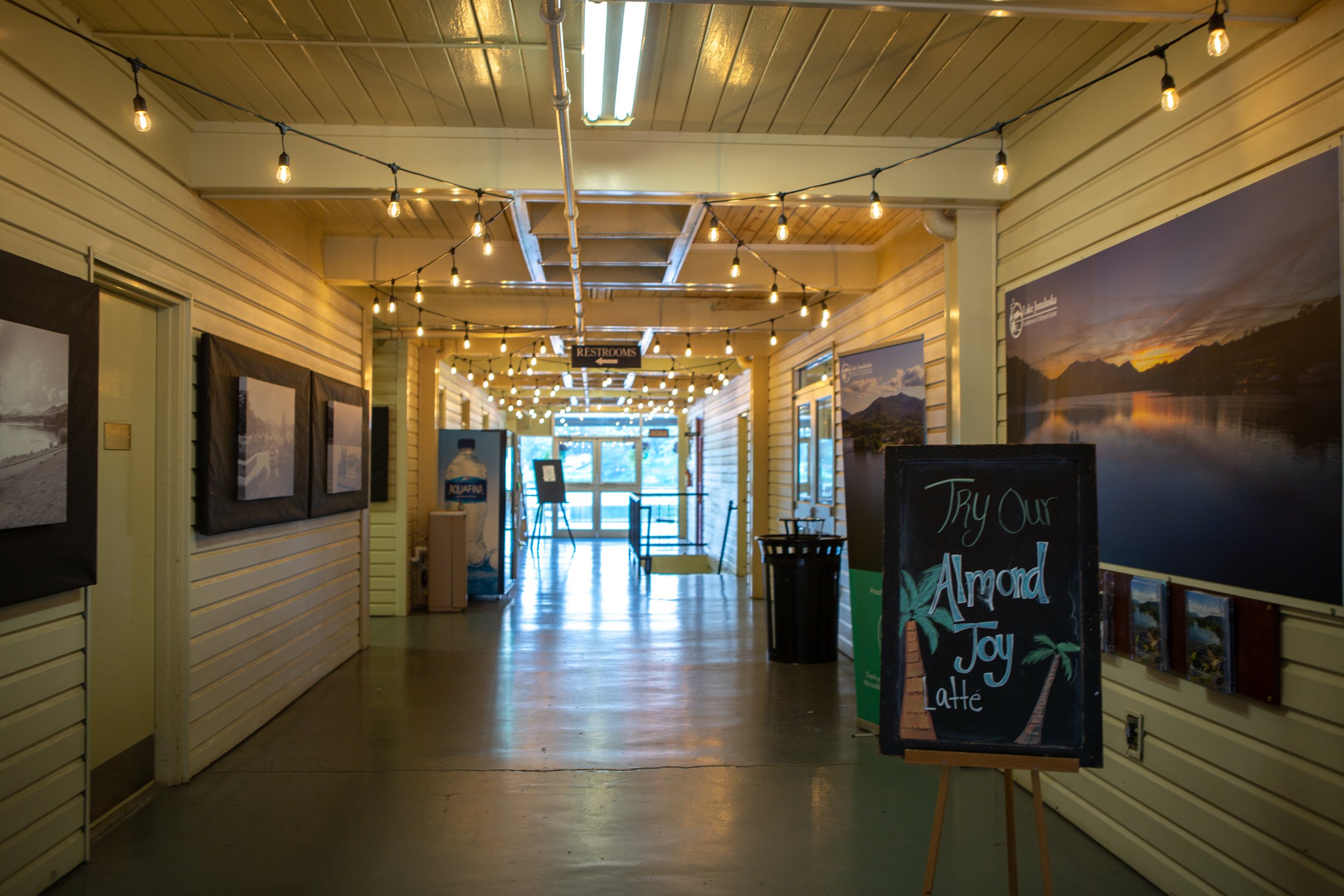The photograph captures the inside of a vibrant, tropical-themed café. The wide hallway is lined with yellowish-tan painted paneling that resembles wood, creating a warm and inviting atmosphere. The ceiling is adorned with string lights and tube lights, adding a cozy glow to the space. Various paintings of landscapes decorate the walls, enriching the environment with scenic art. 

In the foreground, a prominent blackboard sign on an easel stands out. Written in colorful chalk, it invites patrons to "Try Our Almond Joy Latte," with "Almond Joy" and "Latte" in baby blue, and "Try Our" in a vivid yellowish hue. The sign is artistically decorated with hand-drawn palm trees, enhancing the café's tropical vibe.

Further down the hallway, a glass door serves as an exit, with a vending machine featuring an Aquafina advertisement situated to the left. A sign hung from the ceiling directs towards the restrooms, pointing left, and there's a trash can placed in the middle ground on the right. The overall scene is set on a gray concrete floor, contributing to the casual and relaxed ambiance of the café.